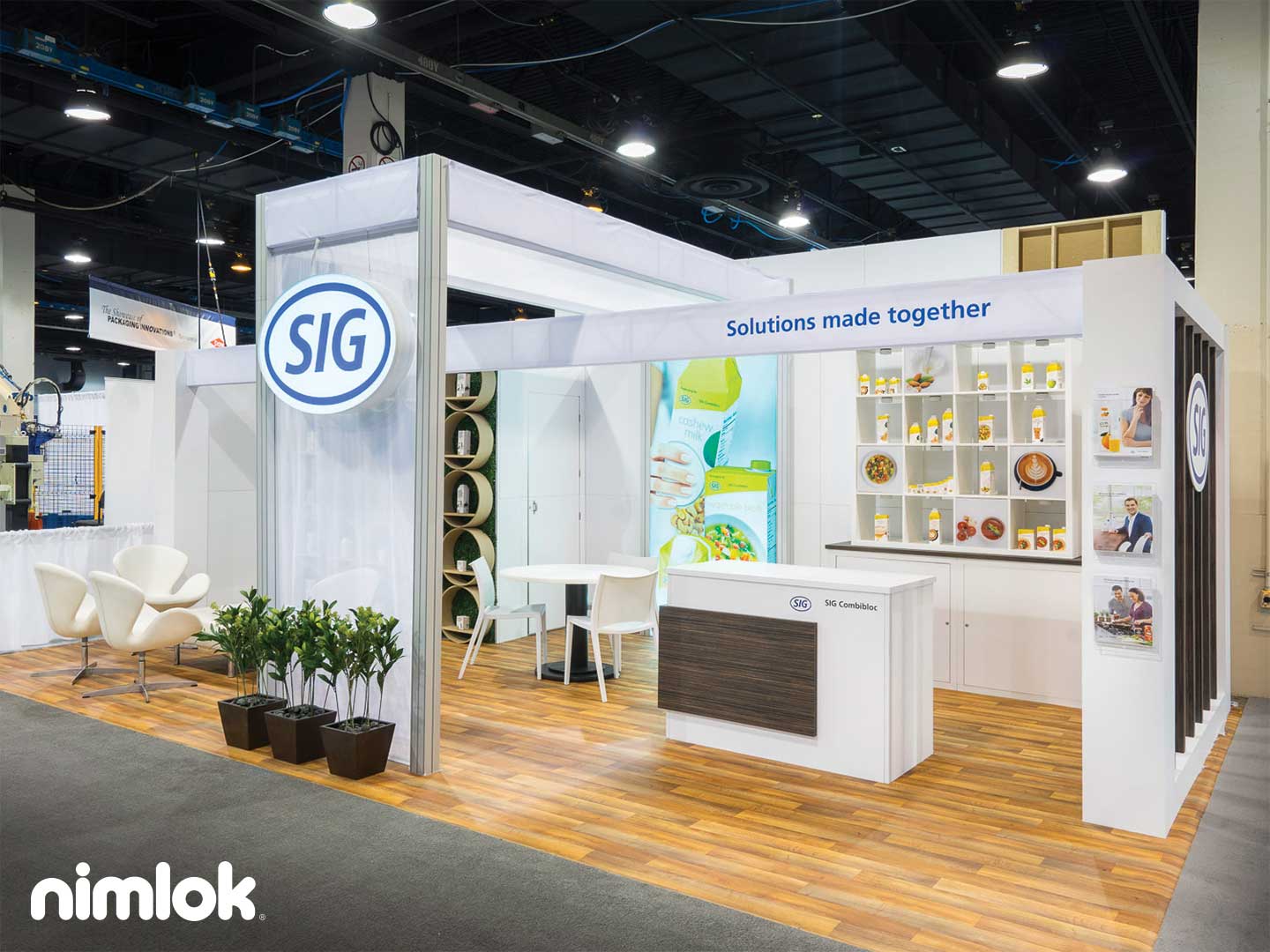The image captures a section of a convention hall or warehouse set up for a presentation or event showcasing various products and innovations. The focal point is a branded display area by SIG, prominently marked with the initials "SIG" in blue letters set within a white circle with a blue outline. This setup features a kitchen display complete with a hardwood floor, a counter, and shelves housing yellow-capped spray bottles. Above the display, a white beam with the message "Solutions Made Together" in blue text spans across the space. To the left, a white banner with a blue top and the phrase "Something Packaging Innovations" is visible. The room's infrastructure includes a ceiling framed in black metal, with rows of fluorescent or halogen lights. Interlocking makeshift walls delineate the display areas, and the surrounding carpet is gray. A table with two chairs and a white bar, labeled "Nimlok," are arranged for attendees to interact with the exhibit.